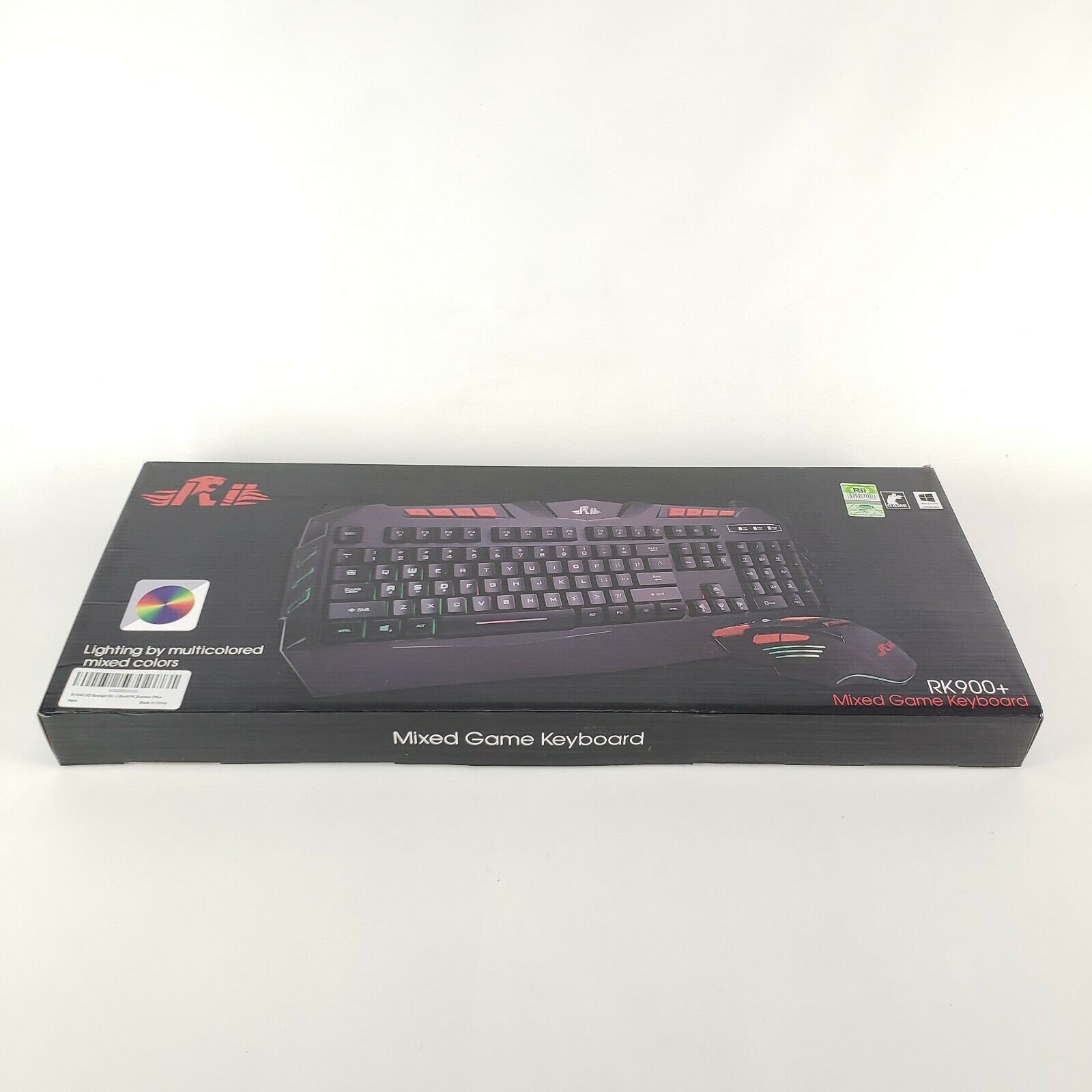This photograph showcases a gaming keyboard presented within its packaging, likely sourced from a website. The keyboard is encased in a predominantly black box that occupies the central area of the image. In the upper left-hand corner of the box, there appears to be a company logo featuring a stylized "R" and "I" with flames on either side, although the exact design is unclear. Below the logo, a color wheel is displayed, indicating customizable backlighting options. The accompanying text, in white, reads "Lightning by multicolored mix colors," suggesting that the keyboard features multiple backlight color selections. A barcode is positioned beneath this text.

In the upper right-hand corner of the box are three logos, whose specific details are not identifiable. The bottom right-hand corner of the box contains the model designation "RX 900 Plus" in white font, with the phrase "Mix Game Keyboard" written in red font below it. Central to the image is a detailed picture of the keyboard itself, exhibiting its design and layout. On the bottom right-hand side of the keyboard, an image of a matching wireless mouse is also included, complementing the keyboard's aesthetic and functionality.